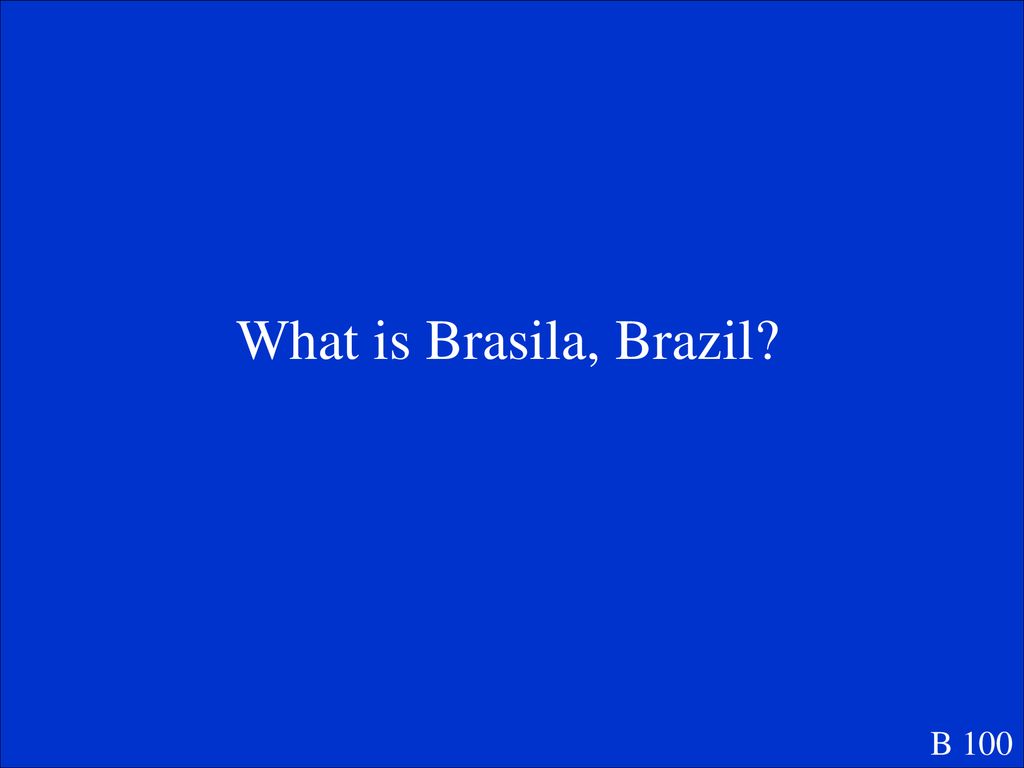The image is a screenshot displaying a computer screen with a bright, vivid blue background that dominates the entire frame. The orientation of the screen is horizontal. At the very center of the image, there's a succinct text displayed in a white font that reads "What is Brazil, Brazil?" with a comma and a question mark. In the bottom right corner, there is a small snippet of text that says "V 100" also in white. The text itself occupies less than 5% of the overall image area, with the rest taken up by the striking blue backdrop. This strong contrast between the blue background and white text creates a visual effect where prolonged viewing makes the letters appear to fade and glow slightly, similar to an optical illusion. There is no visible border or additional details surrounding the text, giving a minimalist and almost hypnotic visual experience.